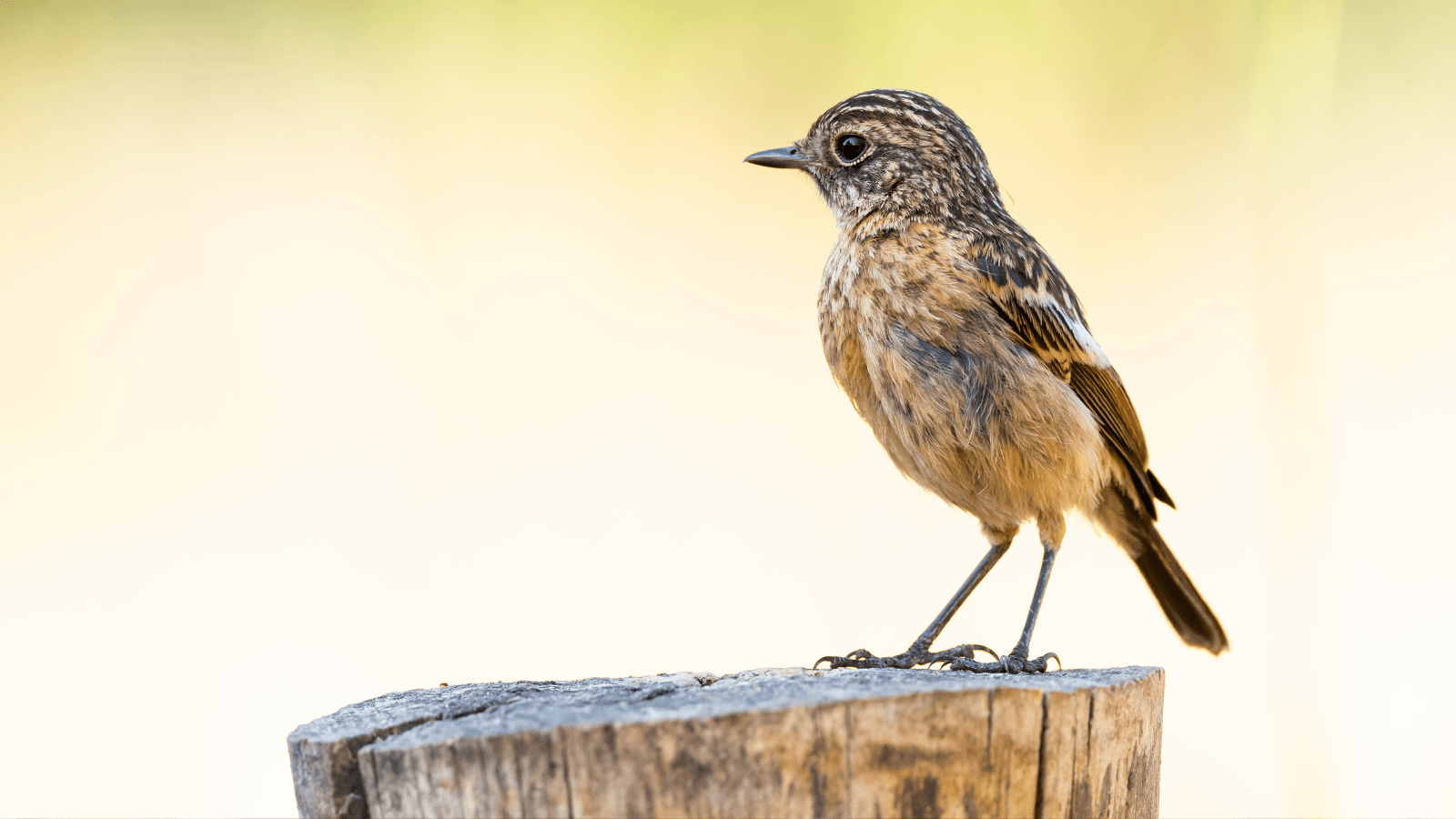The image depicts a small sparrow perched atop a weathered wooden stump, positioned slightly off-center toward the right of the frame. The sparrow, seen in a detailed side profile, features a plumage mix of light brown, dark brown, black, and subtle hints of gray. It has a grey beak and long legs, with black spots peppered across its primarily brown and yellow feathers. The wooden stump beneath the bird displays shades of brown and gray, complementing the bird's earthy tones. The blurred background, transitioning from white to shades of yellow, features subtle hues that suggest a natural, outdoor setting in daylight. The overall style of the photograph emphasizes nature photography, with the sparrow and stump sharply in focus against the softly diffused backdrop.